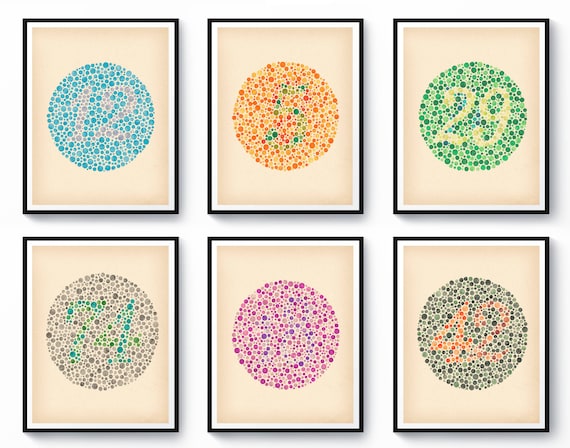The image consists of six framed colorblind test cards arranged in two rows and three columns, all set against a white background. Each frame is bordered in black with a white inner edge, enclosing a tan background. In the center of each frame is a large circle composed of smaller colored dots that form a numerical pattern amidst varying hues.

- The upper left frame features a circle made up of blue and purple dots, displaying the number 12.
- The frame in the upper center showcases an orange and green-dotted circle with the number 5.
- The upper right frame contains a circle of green and light green dots, forming the number 29.
- The lower left frame presents light purple and green dots creating the number 74.
- The center lower frame includes a purple-dotted circle with what appears to be the number 18 in light purple dots.
- The lower right frame consists of green and orange dots, displaying the number 42.

Each number within the circle tests for different aspects of color blindness, using subtle variations in color and hue to reveal hidden numbers.